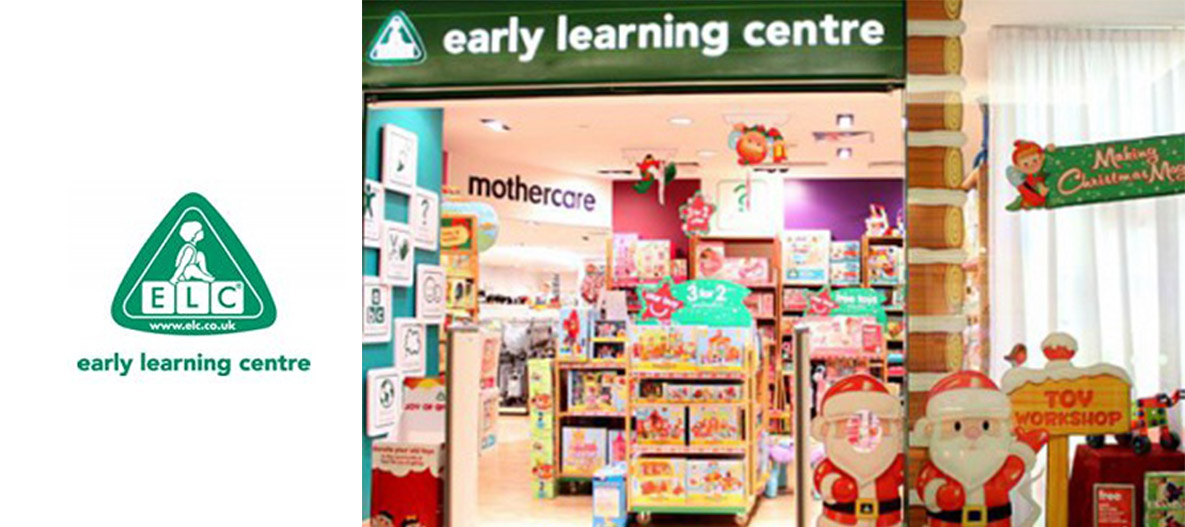This image serves as a promotional advertisement for the Early Learning Center, presented in landscape orientation. On the left side, against a white background, is the Early Learning Center logo: a green triangle with "ELC" printed on white blocks and a woman sitting in profile above, with "Early Learning Center" in green lowercase letters beneath it. Adjacent to this is a photograph depicting the front of an Early Learning Center store. At the top of the photograph is a green banner with the Early Learning Center logo and white lowercase lettering.

In the scene, the store has an inviting holiday-themed display. To the right, a white curtain partially obscures the view, next to which stands a banner with a fairy holding a "Merry Christmas" sign. Below this curtain are a couple of Santa Claus models, standing approximately a couple of feet tall each. There is also a yellow sign reading "Toy Workshop" beside the Santas. The left side of the image shows various colorful aisles and displays filled with toys, though these details are somewhat blurred.

In the background, a wall features the word "Mothercare" in prominent black letters against a cream-colored background, indicating another section of the shopping area. The image captures a moment inside a vibrant and festive retail environment aimed at early learning and childhood development.